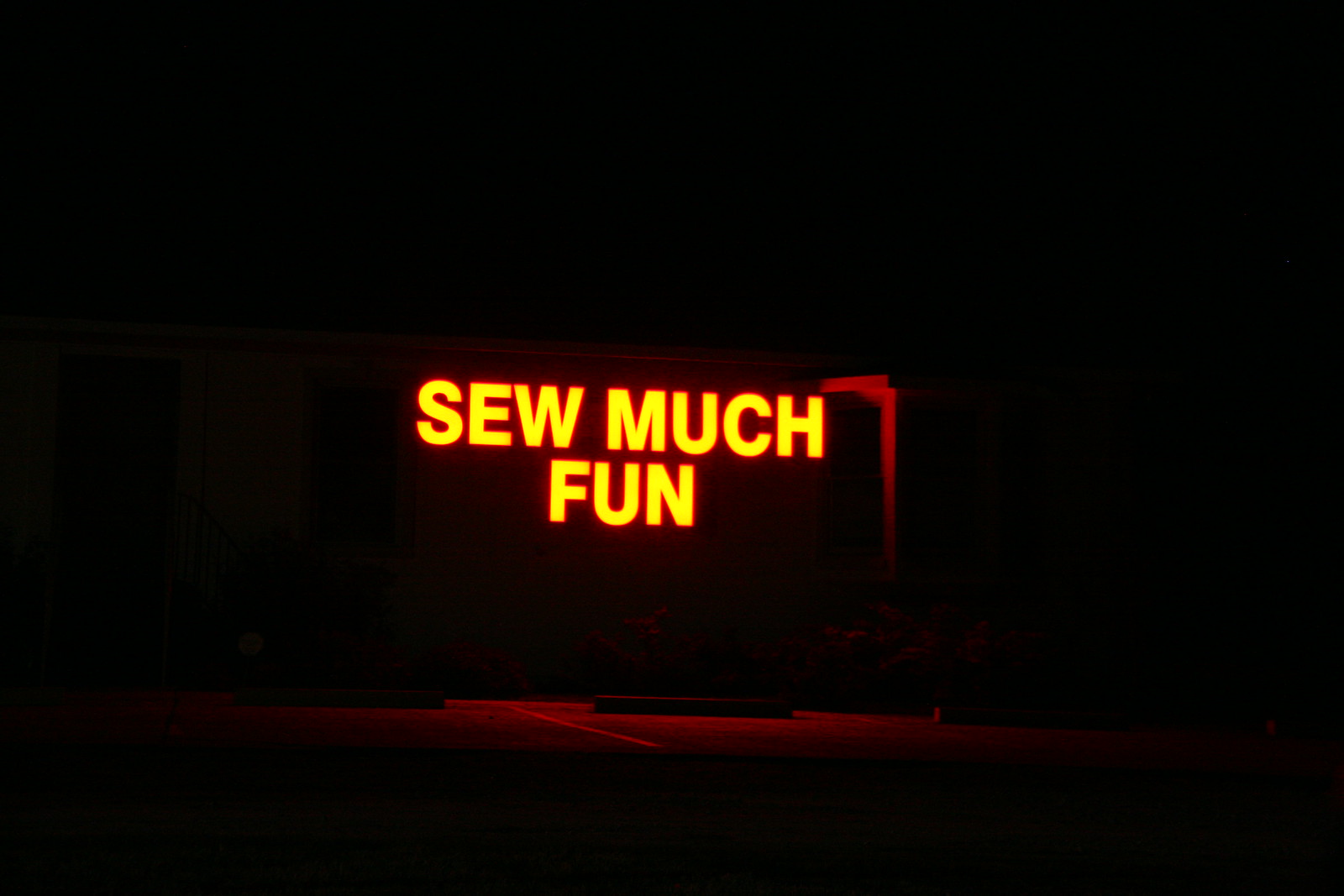In the stillness of night, a vibrant advertising sign for a business illuminates its surroundings against a pitch-black backdrop. The sign, emblazoned with the name "Sue's SEW Much Fun" in bright, attention-grabbing yellow letters, casts a glowing light over the parking lot directly below. The illumination highlights orderly tire stops and clearly defined lines that mark the parking stalls. At the bottom edge of the scene, a sparse brush of bushes softly frames the base of the sign, adding a touch of natural texture to this nighttime tableau.